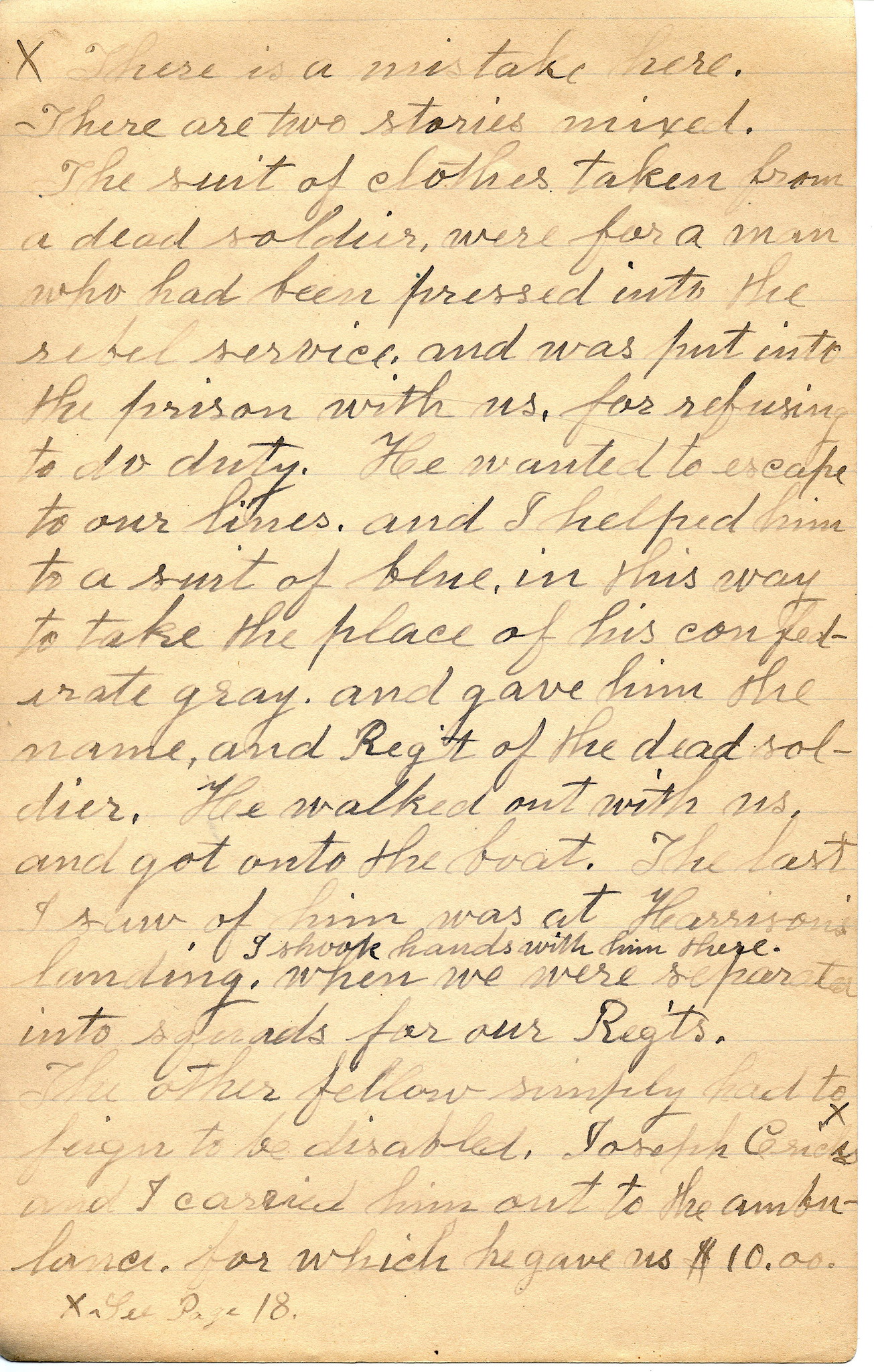This photograph captures a very old, yellowed handwritten letter, showing the wear of time with its off-white, almost brownish paper. The text, meticulously written in cursive with a fountain pen, exhibits a series of dark and fading marks, indicative of the ink drying and being replenished. The letter is composed on ruled notebook paper, faint blue lines guiding the elegant but hard-to-read handwriting. Starting at the top, the letter begins with, "There is a mistake here. There are two stories mixed. The suit of clothes taken from a dead soldier were for a man who had been pressed into the rebel service..." and continues for about 15 more lines. The content of the letter seems to clarify a mix-up regarding a Confederate soldier who was placed into prison for refusing duty and wanted to escape to the Union side. The author recounts how they assisted this man by providing him with a Union uniform, facilitating his escape by helping him assume the identity of a deceased Union soldier. The text paints a vivid picture of wartime subterfuge and personal bravery.